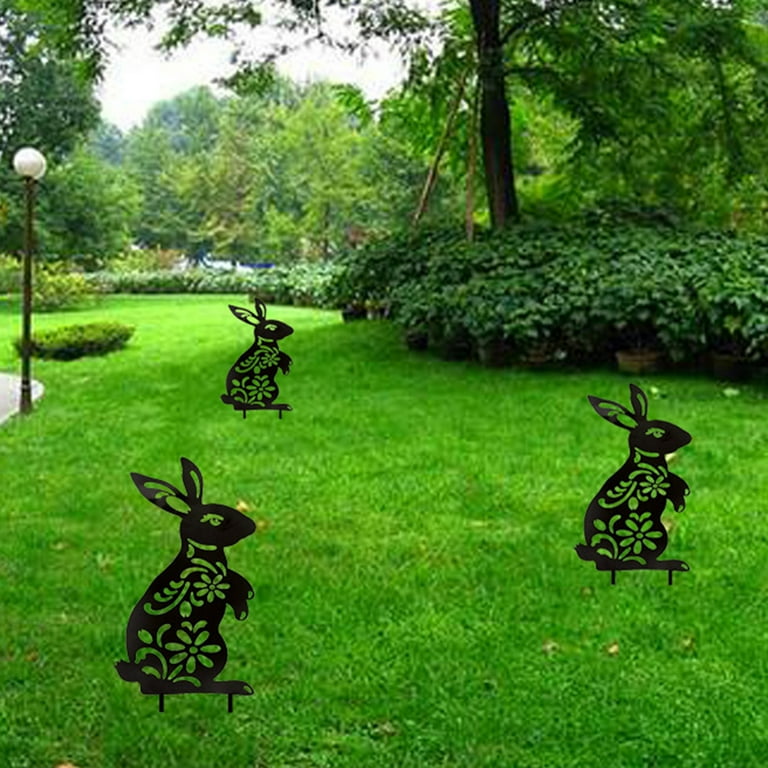This is a detailed daytime photograph of a well-manicured park lawn featuring three prominent flat, black steel rabbit ornaments. These 2D metal rabbit figures are intricately cut with a laser engraver, showcasing patterns that include empty spaces for eyes, parts of the ears, and floral designs. Each rabbit, standing between one and a half to two feet tall, is staked into the vibrant green grass with two spurs. Spread out by several feet, the rabbits add an artistic flair to the already picturesque scene. On the far left, a quaint sidewalk lamppost stands beside a partially visible path, enhancing the park-like ambiance. Surrounding the rabbits is a carefully maintained landscape with potted plants, bushes, and small shrubs, transitioning into a dense backdrop of trees and underbrush, completing the serene and slightly hazy daytime atmosphere.